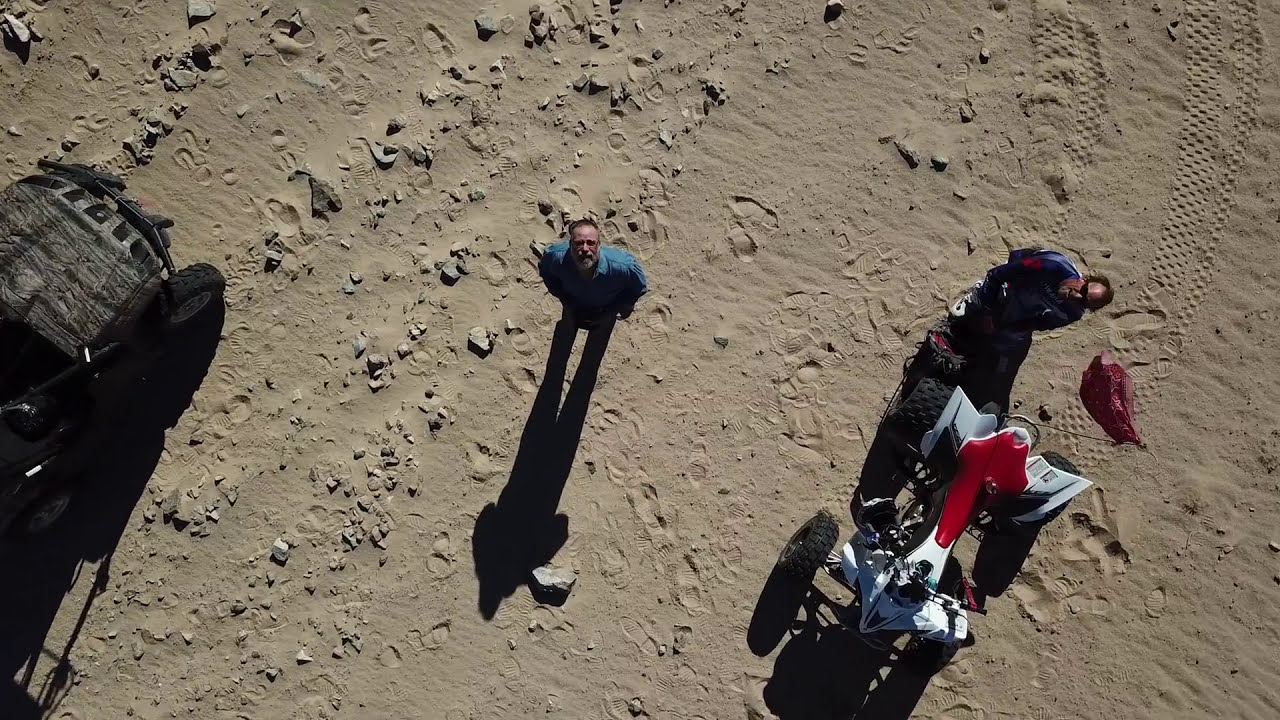From a high vantage point, possibly captured by a drone, the image reveals a sandy and rocky terrain illuminated by the daytime sun. Centered within the frame, an older man with a gray or white beard and donning a blue button-up shirt gazes up at the camera with a puzzled expression. To the left edge of the image, the front end and passenger side door of a camouflaged vehicle, its shadow cast on the ground, are partially visible. To the right of the central figure, another man also looks up, wearing a navy blue jacket and black sunglasses. Directly beneath him sits a white ATV with a red seat, its tire tracks faintly marking the sand. Beside this ATV, a mysterious purple fabric lies on the ground. Both men's shadows stretch across the sandy expanse, emphasizing the bright daylight conditions under which the photograph was taken.